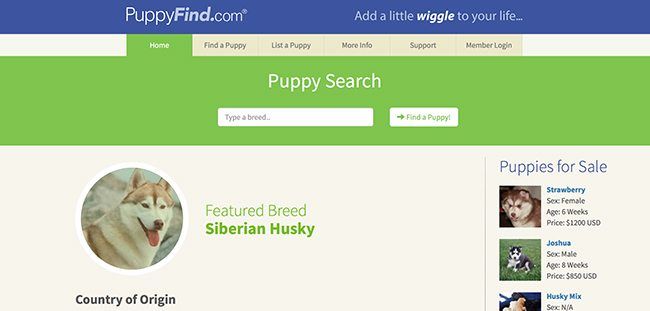This image is a screenshot from a website called puppyfind.com, displayed in landscape mode. The bottom of the image is white and blank, likely indicating it was viewed on a smartphone turned sideways, or possibly on a laptop screen with the bottom cropped off. At the top of the image, there is a navy blue bar with the text "puppyfind.com" in white. The word "find" is italicized, and there appears to be a small symbol, possibly an asterisk or a registered trademark, next to "puppyfind.com." Adjacent to this, the phrase "add a little wiggle to your life..." is displayed, with "wiggle" in white and italicized, and the rest in light blue.

Beneath this heading, there are six navigation tabs. Five of these tabs are tan with black text: Find a Puppy, List a Puppy, More Info, Support, and Member Login. The selected tab is green with white text and labeled "Home," suggesting it either defaults to this tab or the user has selected it. The Home tab opens up a section titled "Puppy Search," featuring a search bar prompting users to "Type a breed," and an associated search button labeled "Find a Puppy." Currently, the breed field is empty, but it defaults to showing results for "Siberian Husky."

Underneath the green Puppy Search bar, a light gray box spans the screen. Inside this box, there is a white-outlined circle displaying a photo of a Siberian Husky. Beneath the photo, it says "Country of Origin," though the specific details are cropped off. Next to the photo, in green text, it states "Featured Breed: *Siberian Husky,*" with "Siberian Husky" in bold.

To the right, a column titled "Puppies for Sale" (in blue text) showcases thumbnail images of three puppies. The first puppy is named Strawberry, a six-week-old female priced at $1200 USD. The next puppy is named Joshua, a six-week-old male priced between $600 to $850 USD; his image shows a black and white dog lying on green grass. The third listing, a Husky Mix, is partially cropped, making the photo and details unclear. It mentions "6N/A" which may suggest multiple puppies.

The image concludes with a sentiment urging viewers to "Adopt, Don't Shop," emphasizing the importance of adopting animals from shelters over buying from breeders.